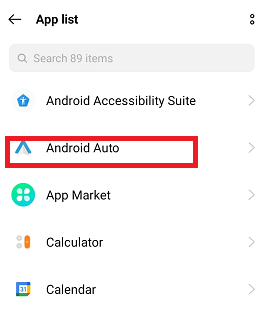In the top left corner of the screen is a small black arrow pointing left, labeled "App List," followed by two small vertical dots. Below this header is a search bar with a light gray placeholder text that reads "Search 89 items." The main content starts with an image of a blue diamond, which is labeled "Android Accessibility Suite." 

Underneath this, a red-outlined square contains an icon of a blue arrowhead pointing upwards accompanied by the text "Android Auto." Next, a blue circle with four small white dots inside symbolizes the "App Market." 

Following this is an icon consisting of two small dots and a long orange circle labeled "Calculator." Further down, a boxed icon with a combination of blue, yellow, and green colors features the number "31" in its center, and about two inches to the right is the word "Calendar," spelled out in black as "C-A-L-E-N-D-A-R." 

The primary focus here is on the red-outlined area highlighting the "Android Auto" section.